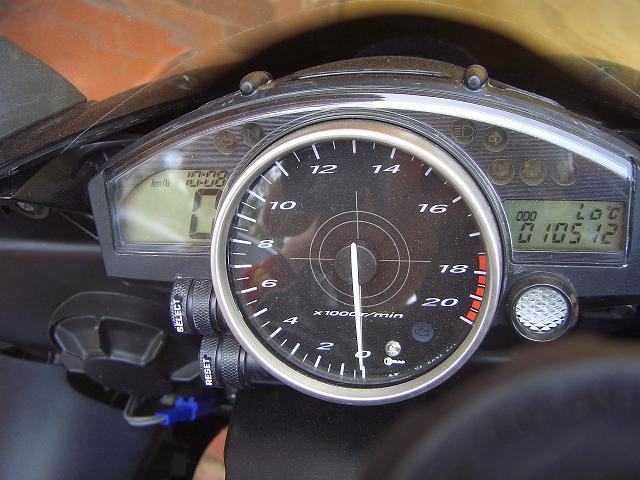The photographic image features a detailed view of an instrument cluster from a vehicle, prominently displaying a round dial. The dial has a black face and a white needle, with measurements ranging from 0 to 20. The dial is marked "x1000/minute," indicating it is likely a tachometer for measuring engine RPMs. Notably, the scale turns red as it moves past 18, signifying a warning or danger zone towards 20. 

On the left side of the dial, there is an indicator displaying "10-0-8," possibly a calibration mark or part number. The instrument panel includes signal lights for left and right turn signals, as well as an indicator for high beams and a neutral gear position. To the right of the main dial, there is another segment marked "0-1-0-5-1-2" and labeled "Low °C," potentially indicating a low temperature warning.

Situated below the main dial is a cap, beneath which you can see buttons labeled "Select" and "Reset" for adjusting the settings or resetting the measurements. Adjacent to these buttons is a white circular light. The entire assembly is part of a single, cohesive piece of dashboard instrumentation.